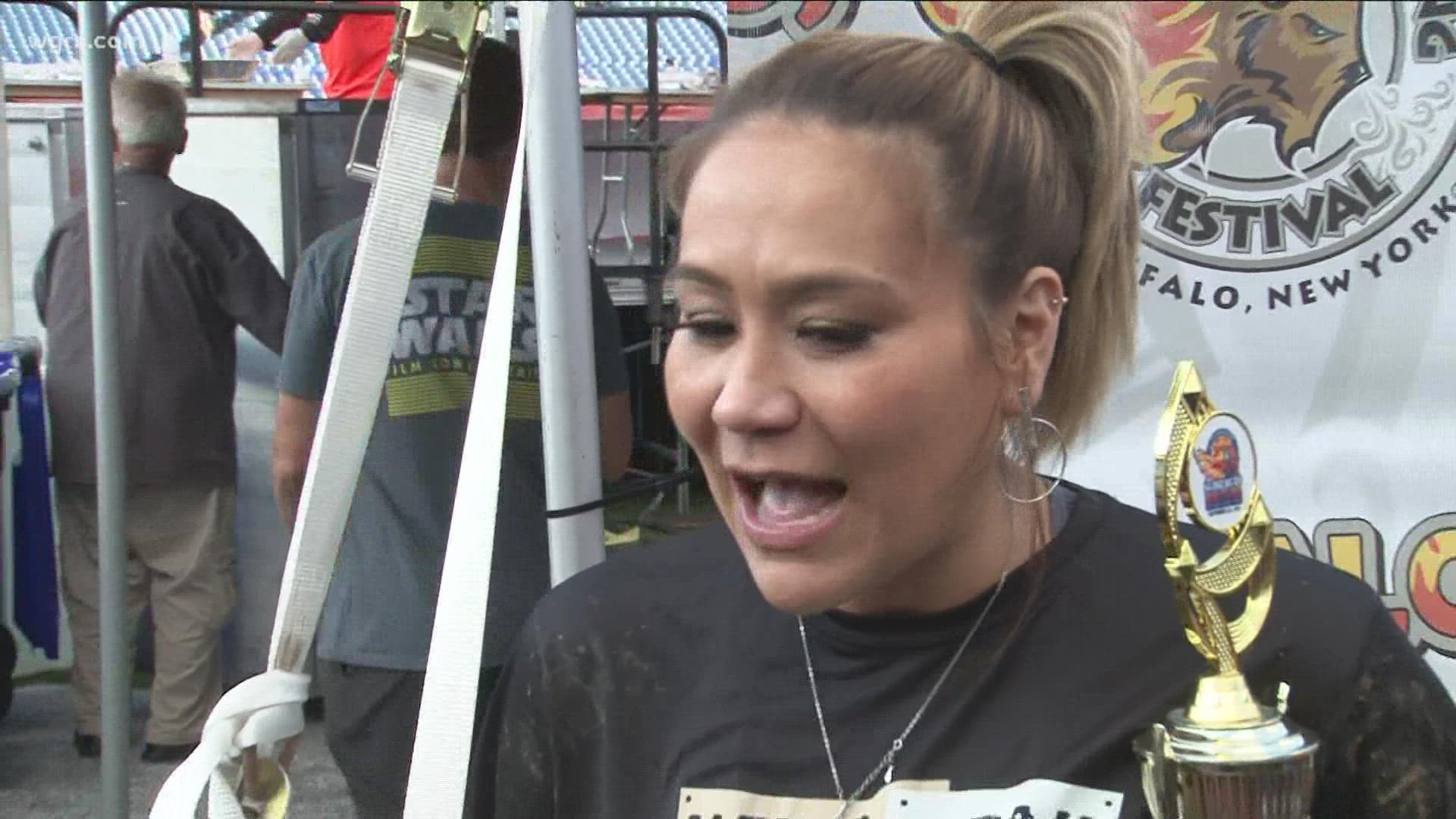In this real-life photo taken at a festival in Buffalo, New York, a Latina woman in her mid-30s is prominently featured in the foreground. She has her hair pulled back into a high ponytail and is adorned with silver hoop earrings, a cuff earring on the upper arch of her ear, and a silver necklace. She's wearing a black t-shirt with a graphic design and appears to be holding a trophy, which she likely won in a buffalo wings contest, either for eating or preparation. Her mouth is open as if she's talking to an interviewer or a camera, though a microphone isn't visible.

In the background, various elements of the festival are depicted, including men who seem to be packing up or cleaning the event area. Among them, one man is wearing a Star Wars t-shirt in gray, yellow, and white, and another older man with white hair is dressed in a gray shirt and gray pants. The backdrop includes tents and banners promoting the Buffalo festival, further emphasizing the setting.